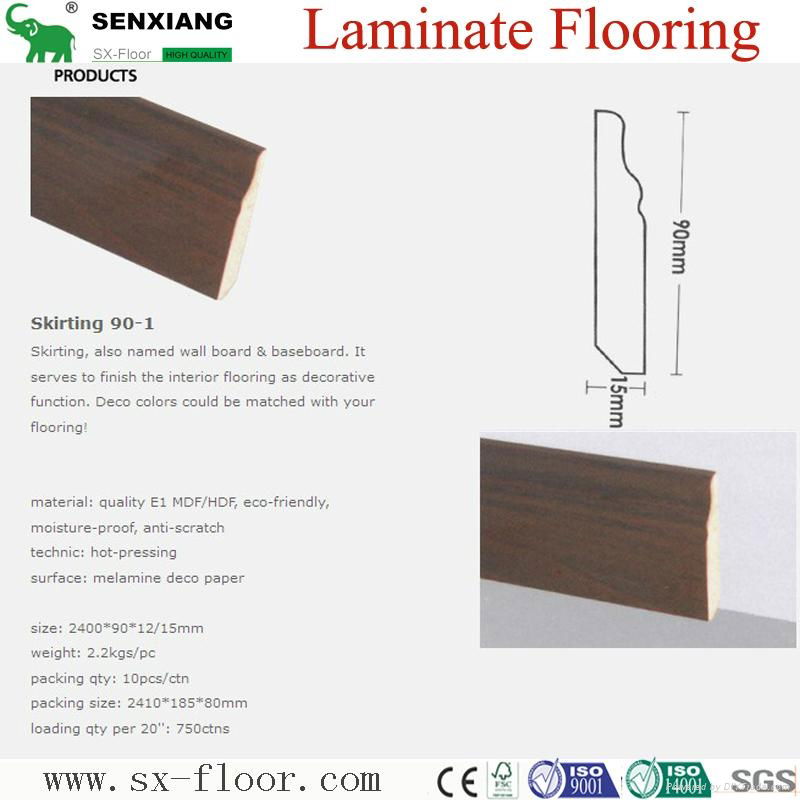The image is a detailed product information sheet for laminate flooring from the company Sen Xiang, characterized by their green elephant logo in the upper left corner. The brand name "SEN XIANG" is prominently displayed in black text beside the logo, with "X-FLORE HI-QUALITY" noted beneath it. Red serif font at the top right declares “Laminate Flooring.” 

The sheet includes a detailed description of a product called "Skirting 90-1," which is also known as wallboard or baseboard. This component serves both as a decorative and functional element finishing the interior flooring. The image displays a dark brown piece of baseboard, highlighting its ability to match various deco colors.

Key specifications include: 
- Material: Quality E1 MDF/HDF, eco-friendly, moisture-proof, and anti-scratch.
- Technical details: Hot pressing surface with melamine deco paper.
- Size: 2400 x 90 x 12 and 15 millimeters.
- Weight: 2.2 kilograms per piece.
- Packing: 10 pieces per carton, with a carton size of 2410 x 185 x 80 millimeters. 
- Loading capacity: 750 cartons fit in a 20-foot container.

Additional visual elements include a schematic outline of the skirting dimensions and another product image. At the bottom of the image, the website www.sx-floor.com is displayed, accompanied by certification logos such as CE, FSC, ISO 9001, ISO 1401, and SGS, underscoring the product's compliance with industry standards. The background of the sheet is primarily grey with thin white borders at the top and bottom.